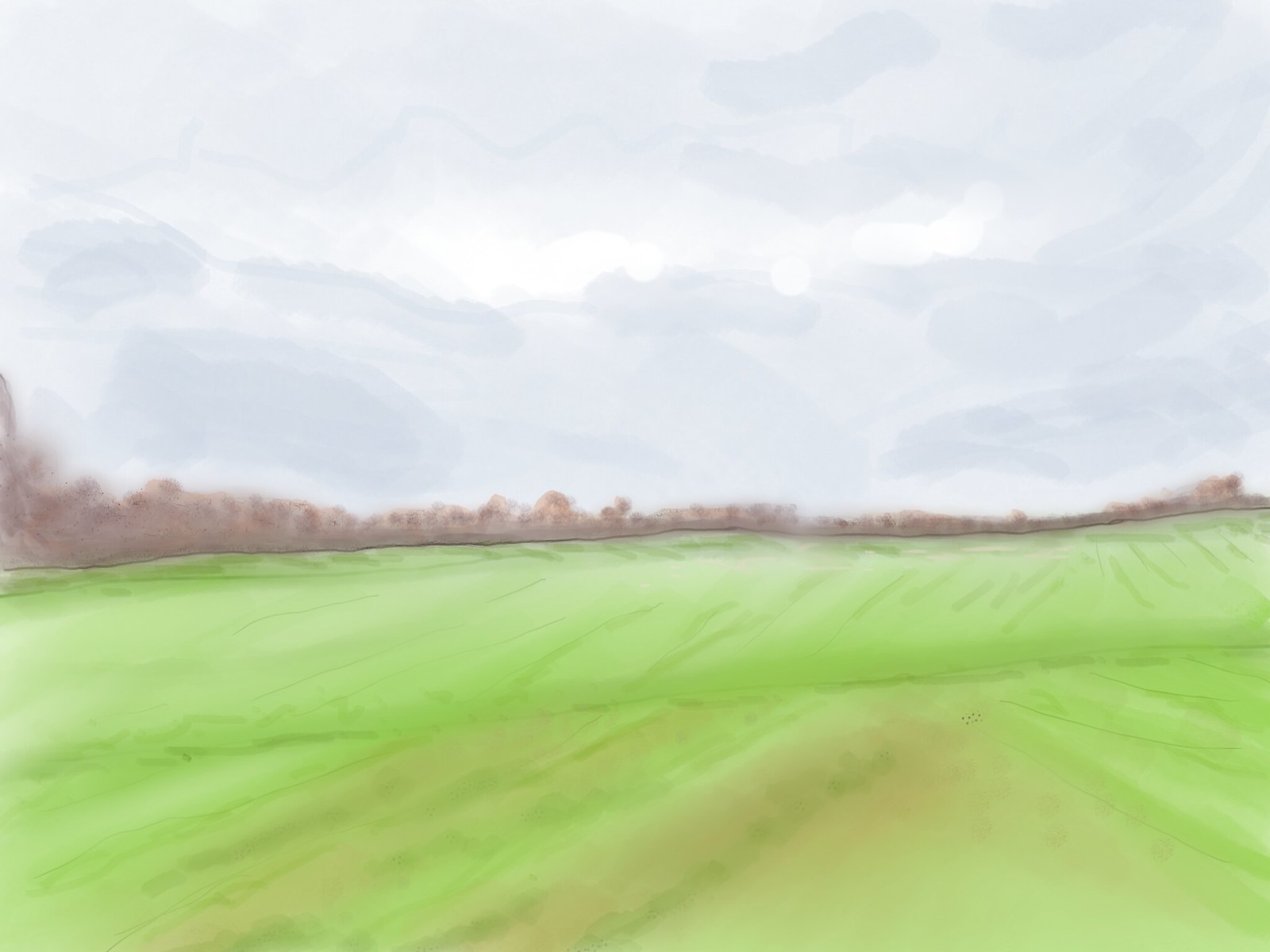This detailed painting is a surrealist landscape characterized by its ethereal, watercolor-esque appearance. Dominated by varying shades of green, the foreground features flat, bright green grass that fades to near-white in places. Dried-out trees, depicted in light and dark browns, dot the scene, adding texture and contrast. The sky above, filled with fluffy, grayish-white clouds, stretches across the canvas with visible large brush strokes and wavy lines. The blending of gray and white paint creates a soft, dreamy atmosphere, further enhanced by the occasional white streaks that appear toward the center of the painting. Overall, the image combines elements of the real and the surreal, with its blurred details and rich, varied colors, creating a strikingly surreal and ethereal aesthetic.